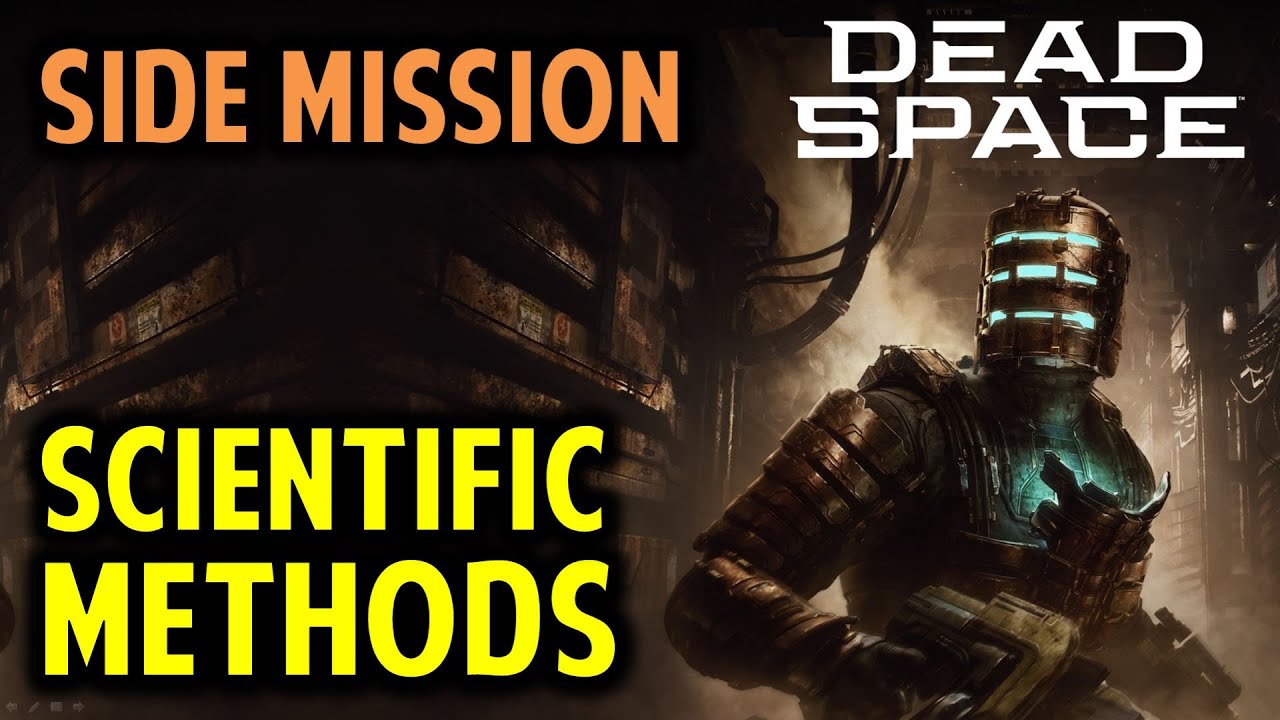The image is a promotional banner for a video game, featuring dark, dystopian digital artwork with a futuristic theme. The banner itself is rectangular, with a length twice as long as its width. In the top left corner, bold orange text reads "SIDE MISSION," while the bottom left corner features bold yellow text stating "SCIENTIFIC METHODS." In the top right corner, bold white text with a partially missing 'E' reads "DEAD SPACE." The bottom right corner showcases a character in a detailed, futuristic bronze-colored space suit, complete with light blue glowing accents. The character's helmet, reminiscent of medieval armor, has three illuminated slits across the faceplate, and his body armor is segmented with a prominent, glowing blue light on his chest. The background depicts a ruined, dystopian city shrouded in smoke, enhancing the dark atmosphere of the image.